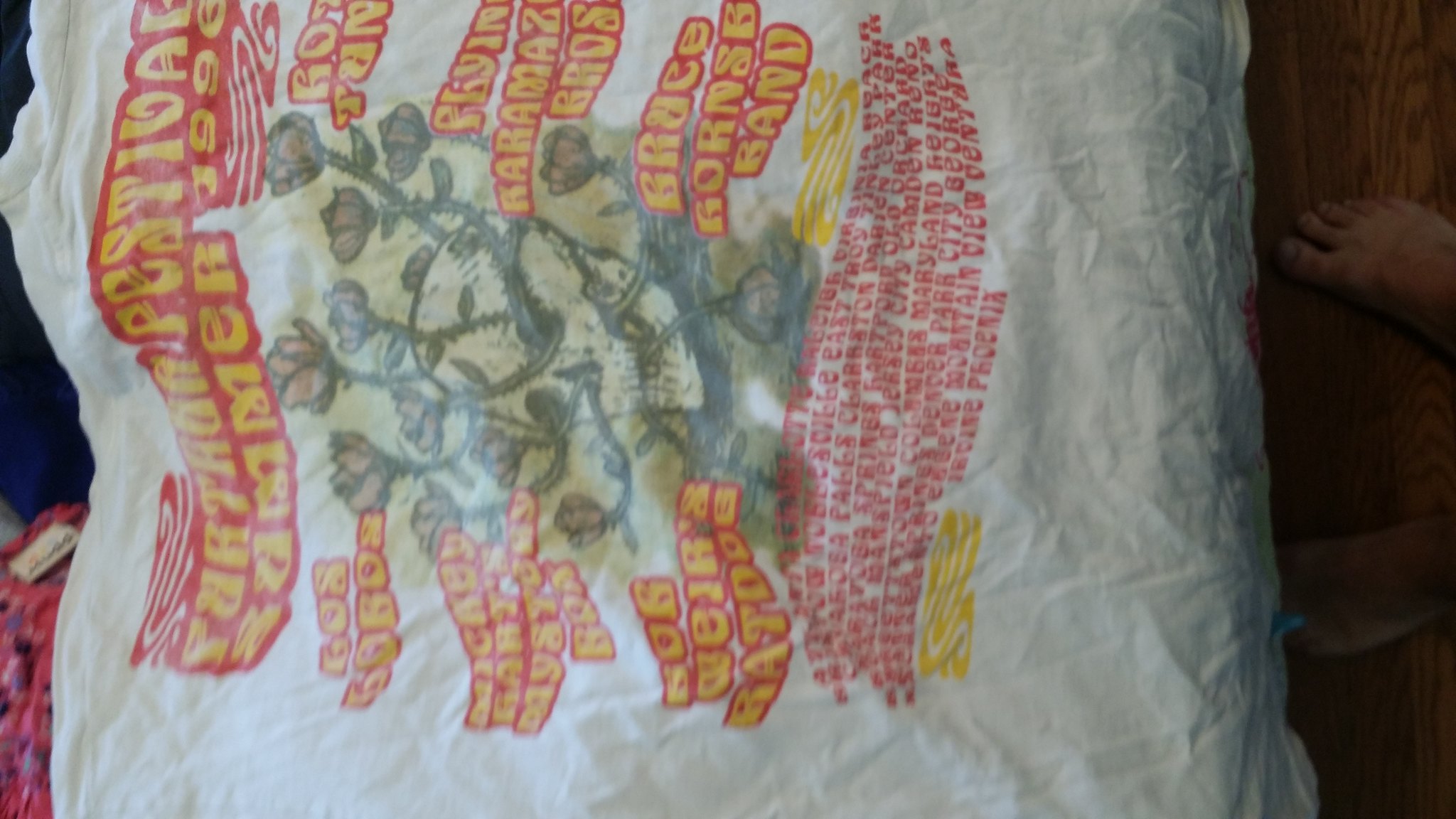This captivating image showcases a crinkled white T-shirt sprawled horizontally on a wooden floor. The focal point of the T-shirt is a vividly colored plant motif in the center, resembling a delicate flower. Surrounding this central floral graphic is bold text with a striking design: the left side features red outlined letters filled with yellow, while towards the right side of the T-shirt there are small lines of red text. The entire composition is accentuated by the presence of someone's feet on the right side of the frame, adding a touch of human element to the scene. This delightful juxtaposition captures the essence of casual fashion and homey tranquility.